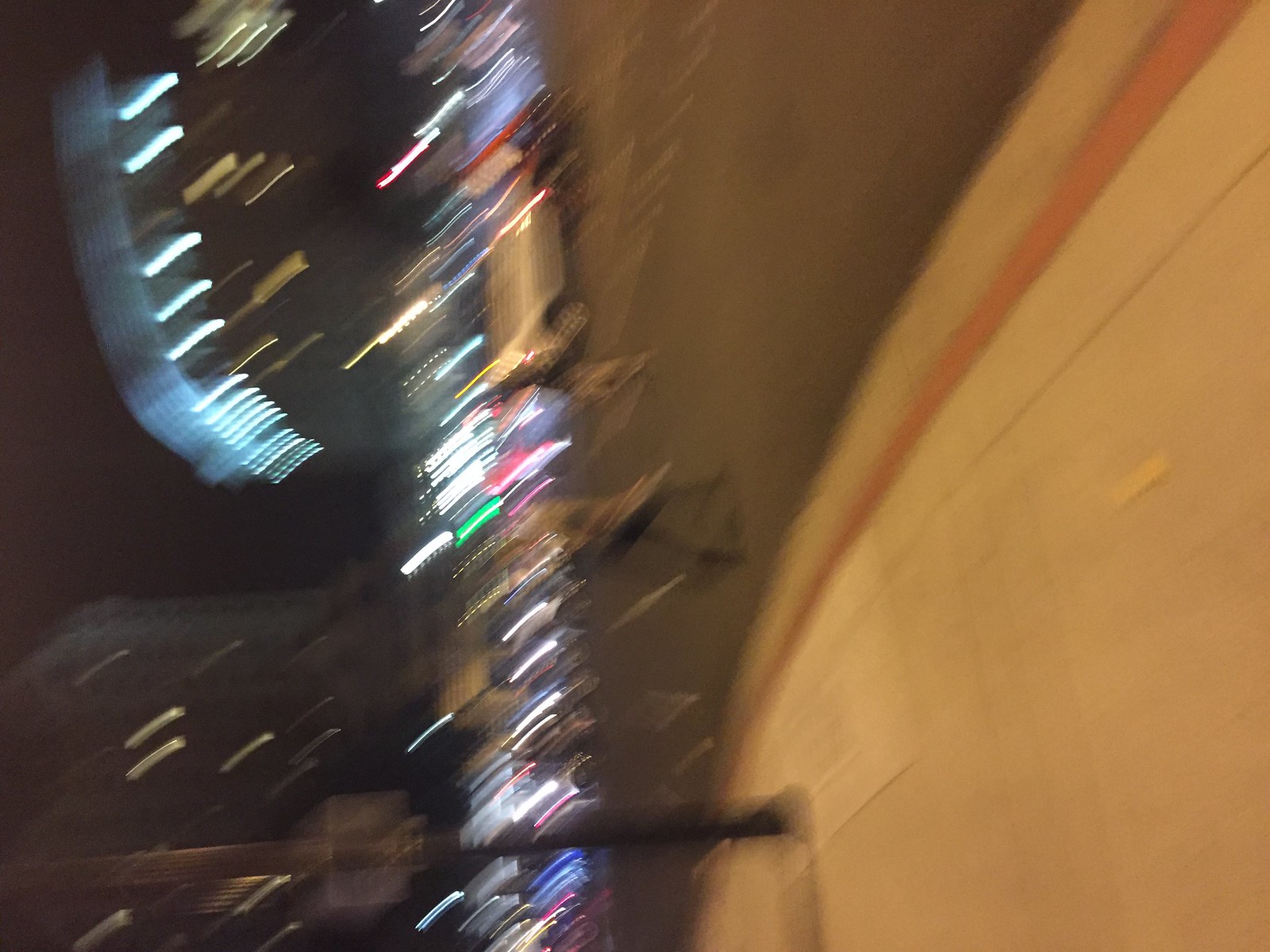The photo appears to have been taken during a very drunk night out, likely accidentally while walking with the phone in hand. The image is a blurry color photo, showing a scene that is difficult to discern due to significant motion blur and poor lighting. The pavement, visible but turned sideways, suggests the camera was swinging, possibly creating a slow exposure effect. Bright, colorful lights from cars—appearing as horizontal stripes in blue, white, green, darker blue, and red—add to the chaotic feel. There's also a somewhat discernible lamppost, which is horizontal rather than vertical. However, everything is incredibly blurred, including a car in the background and what might be people walking. The scene's movement and light distortion make it look almost like an abstract, arty photo, with elements that could suggest being in a tunnel, indicated by glimpses of a white tiled wall, an asphalt road, and a ceiling with possible piping.